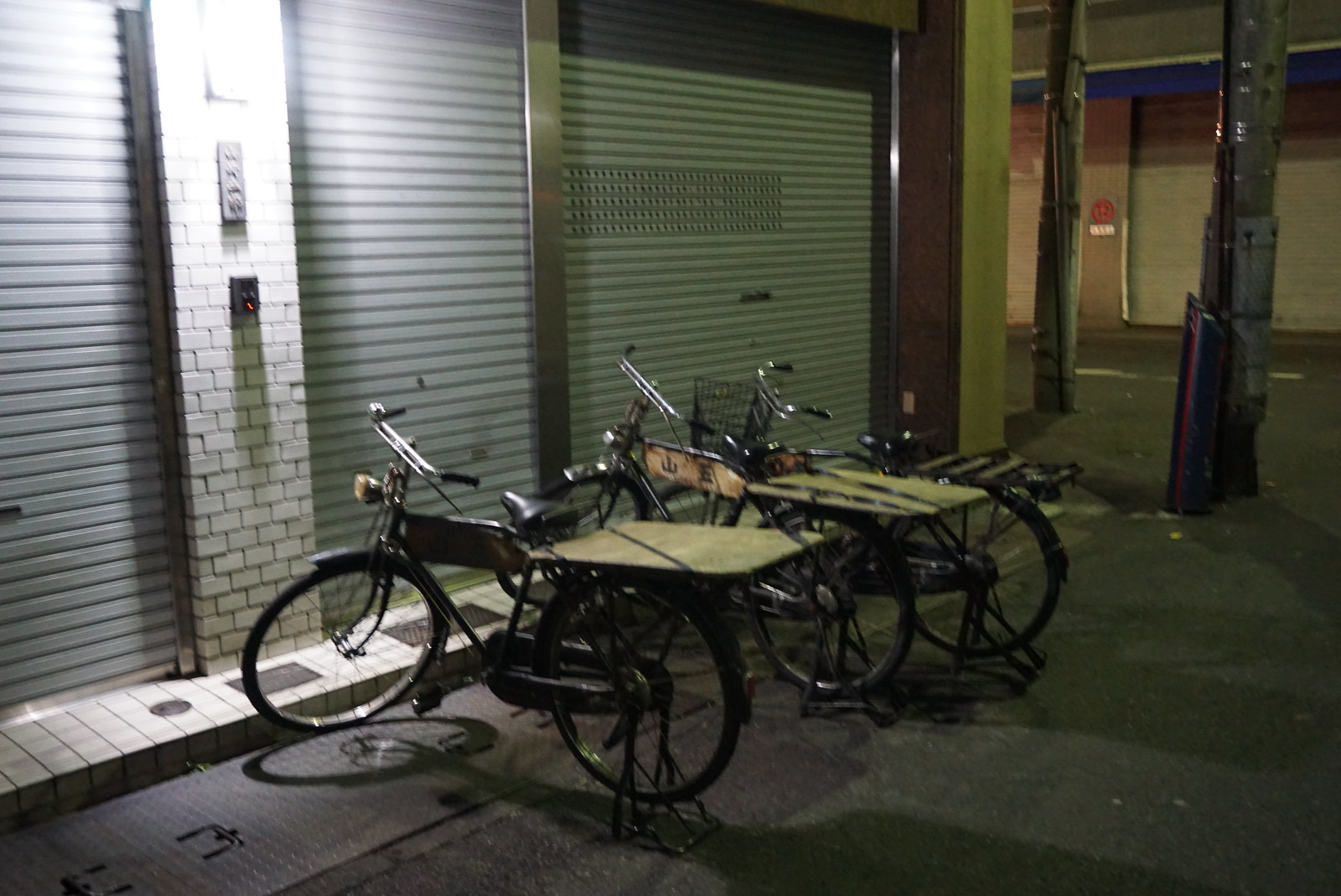This nighttime city street photo is centered on three black bicycles, likely used for deliveries, each equipped with headlights and wooden back platforms. The bikes are parked on a concrete area in front of large, silver corrugated metal garage doors, illuminated by a light above. These garage doors are trimmed with metal, and a distinct brick column with a red-lit black device is partially visible on the left side. The photo captures the surrounding urban setting, showing some white brick and parts of an older, possibly unoccupied building with large windows in what looks to be an alleyway. To the right edge, the street and a couple of telephone poles are also noticeable, adding to the cityscape's ambiance.